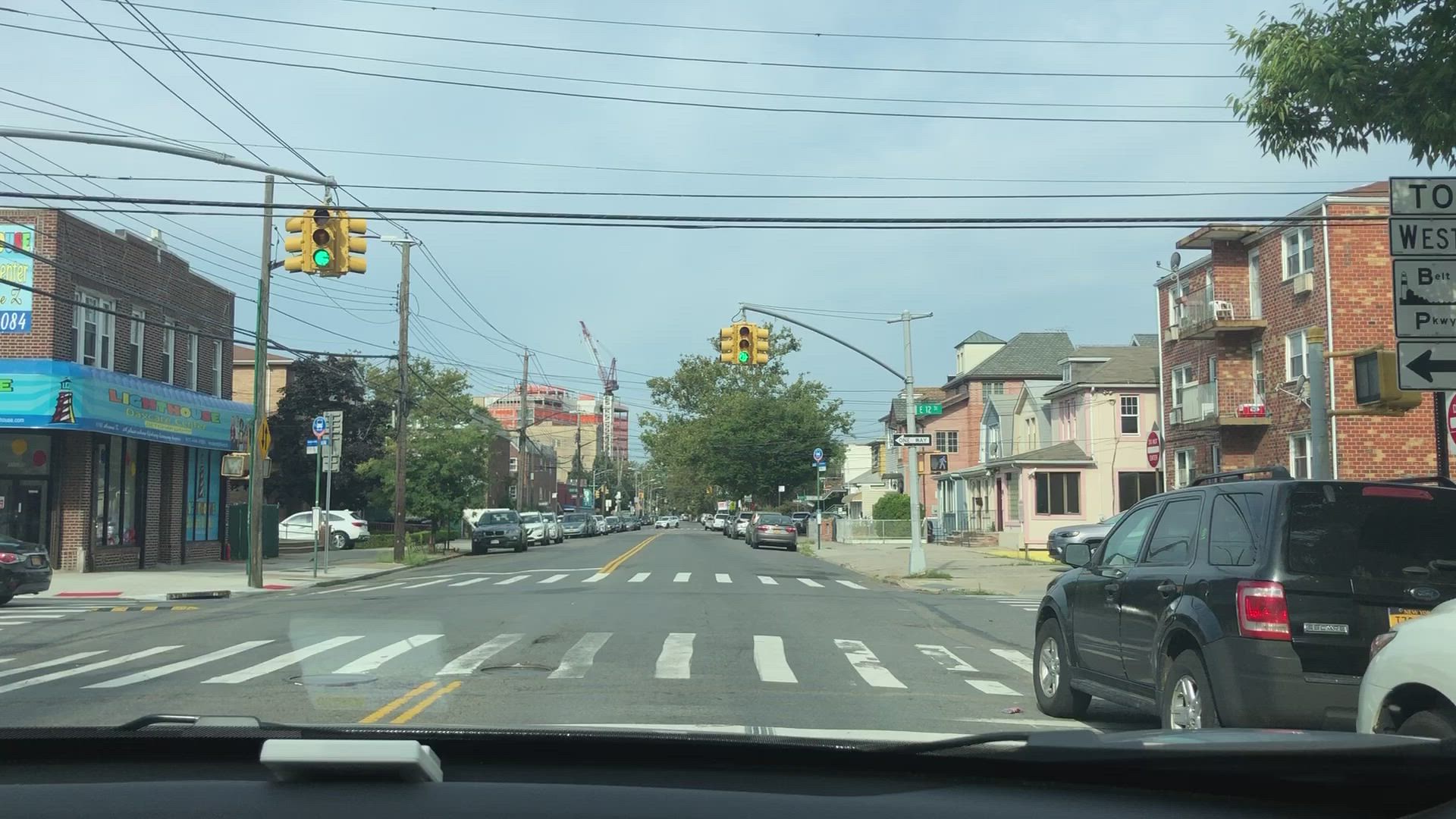A bustling residential street lined with parked cars stretches into the distance. On the right side of the street, a mix of apartment buildings and smaller houses form a diverse urban landscape. Prominently, a street sign mounted on a light pole indicates "East 12th Street" with a one-way arrow. Another light pole on the left side of the street also displays a green traffic light. Amidst a variety of street signs, a crane can be seen in the background, contributing to the construction of a larger building. The neighborhood, predominantly residential, features one notable business, "Lighthouse Daycare Center," housed in a brick building with its own parking area. Despite the cloudy sky, the view through the front windshield reveals a clear daytime scene, characterized by an abundance of parked cars and an active street life.